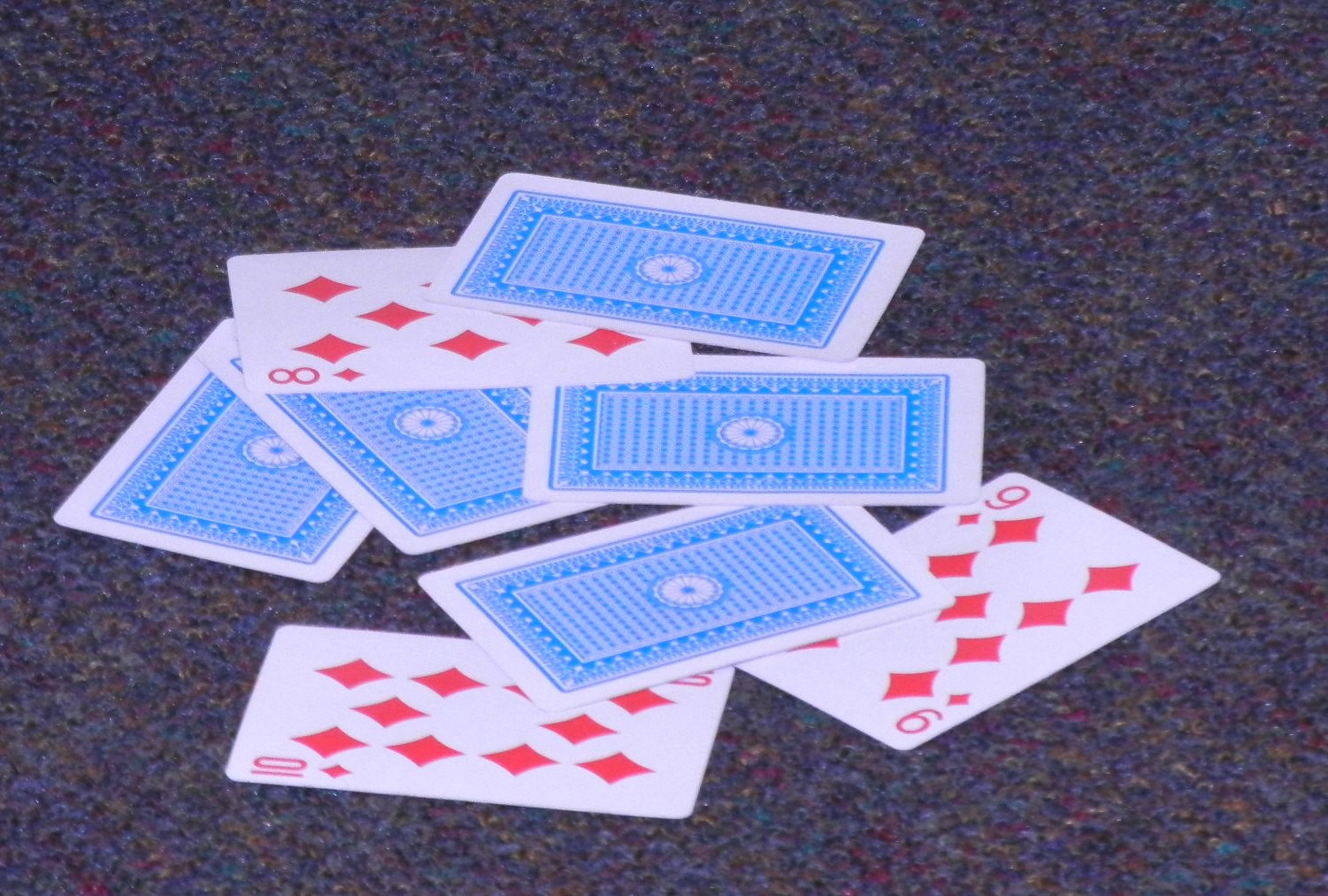The image features an antique, multi-colored wool rug adorned with an array of intricate, woven patterns. The rug showcases a rich tapestry of reds, yellows, purples, blues, greens, and turquoises, creating a visually striking and colorful canvas.

Atop this vibrant rug lies a neatly arranged collection of playing cards. There are eight cards in total, symmetrically spread out. Among these, three cards are face up, revealing the eight of diamonds, the nine of diamonds, and the ten of diamonds. This arrangement invites curiosity about the identity of the remaining five face-down cards, leaving one to ponder whether they too belong to the diamond suit or if their placement is merely coincidental.

The playing cards themselves are distinct with blue and white backs featuring intricate designs. The backs display a circular motif with a small blue dot centered within it, adding to the detailed and ornate aesthetic of the scene.